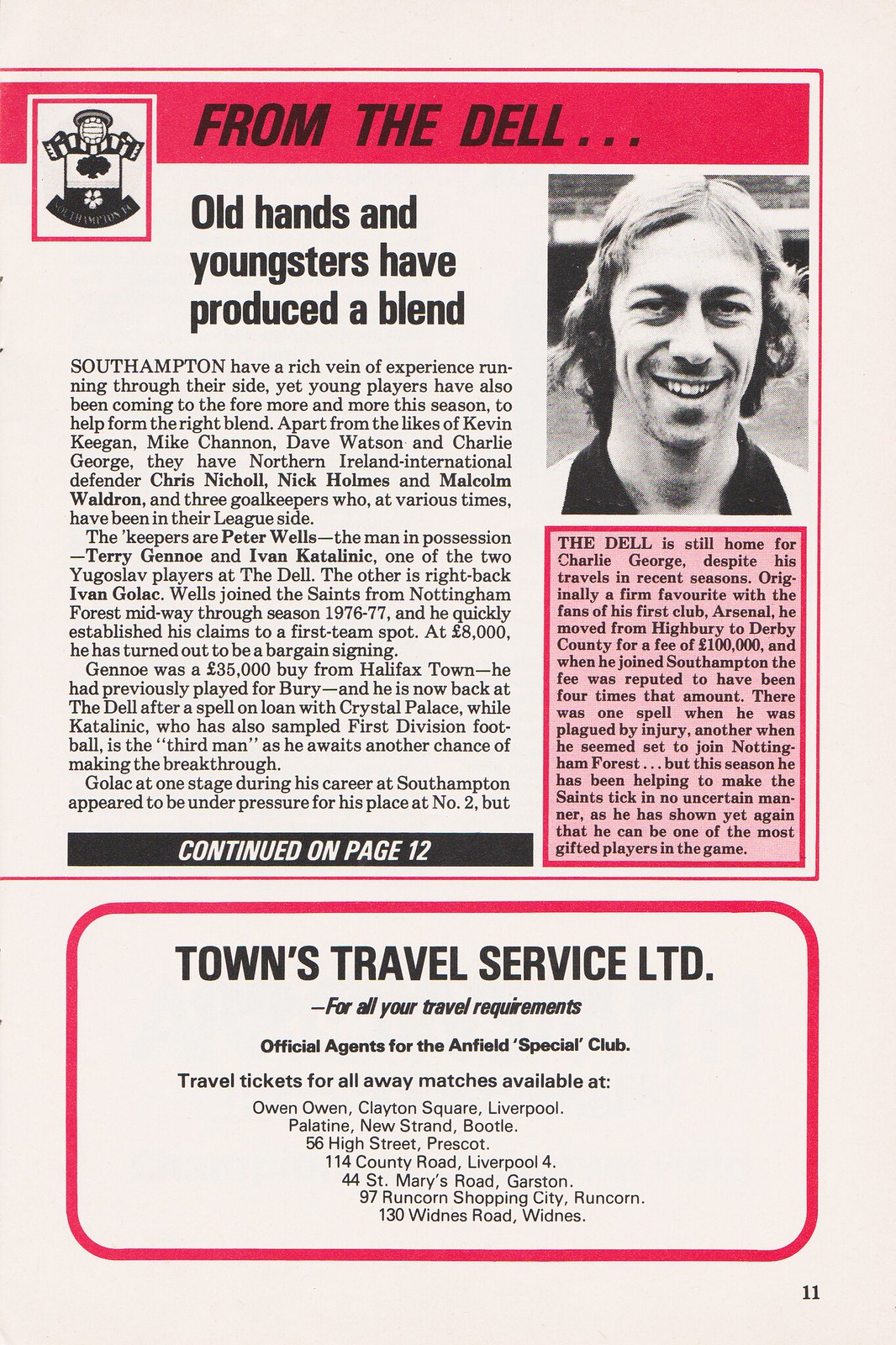This image appears to be a page from a vintage magazine or newspaper, possibly from the 1970s or 80s, characterized by its cream-colored background. Dominating the top section is a distinctive red banner with black text that reads "From the Dell," alongside an emblem, presumably the logo of a soccer club. The focal point is a black-and-white photograph of a young man with a mustache and scraggly hair, smiling, likely a soccer player named Charlie George. Beneath his image, a red textbox with black lettering declares, "The Dell is still home for Charlie George despite his travels in recent seasons," alluding to his career moves which included a notable transfer to Derby County for £100,000.

Adjacent narratives emphasize Southampton's soccer team, juxtaposing seasoned veterans with emerging young players to form a synergistic squad. Text revealing player transactions includes mentions of Kevin Keegan, Peter Wells, Terry Ganneau, and Ivan Ketamine, detailing Ganneau's transfer from Halifax Town for £35,000 and his earlier stint at Barrie. A specific note marks the continuation of this article on page 12.

Towards the bottom, an advertisement in a red-outlined rectangle stands out, promoting "Towns Travel Services LTD for all your travel requirements," identifying them as the official agents for the Anfield Special Club with exclusive travel offers for away matches. The page also shows a small number 11 at the bottom right, indicating its position in the publication.